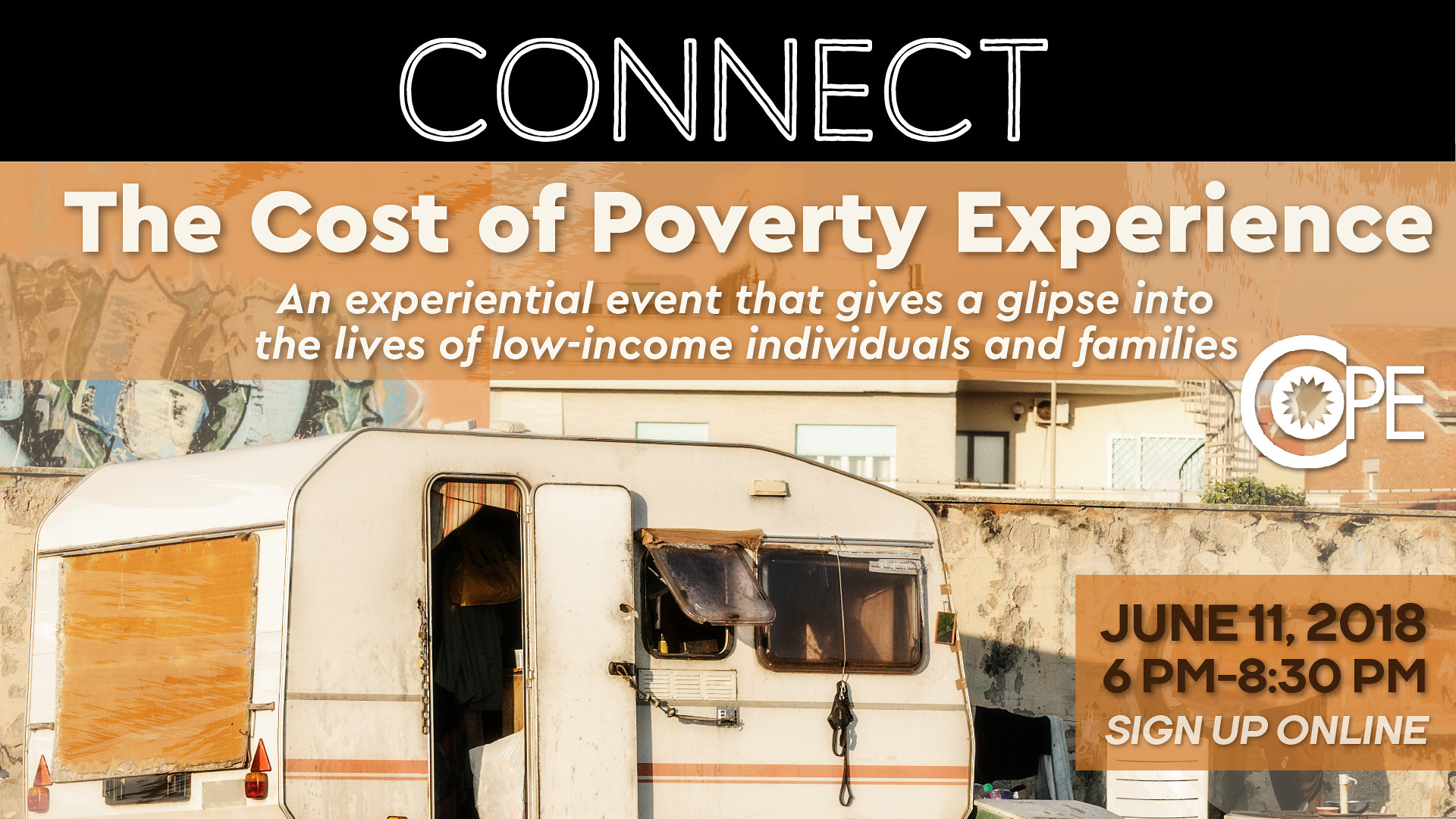The image is an advertisement featuring a detailed poster in landscape orientation. At the top, a black banner houses the word "CONNECT" in bold white outline text. Below this banner, the primary image captures a grungy, rundown RV, with wooden planks covering parts of the windows and visible rust. The RV's dilapidated appearance is contrasted with its background, which includes debris, a dirt-stained wall, and a distant building.

Centrally positioned, the heading "THE COST OF POVERTY EXPERIENCE" in white text highlights an event aimed at providing insights into the lives of low-income individuals and families. Below this, a smaller italicized white text reads, "An experiential event that gives a glimpse into the lives of low-income individuals and families." Notably, the word "glimpse" is misspelled as "glipse."

To the right of the central text, a distinct logo for the organization COPE is displayed. The design integrates the letter "C" encircling an "O" with a sunburst inside, with the "P" matching the size of the "O." At the bottom of the image, event details are provided in black text over a partially transparent orange band: "June 11, 2018, 6 p.m. to 8:30 p.m. Sign up online."

The overall style merges photographic realism of the impoverished RV scene with structured graphic design elements to deliver a poignant and informative visual narrative.